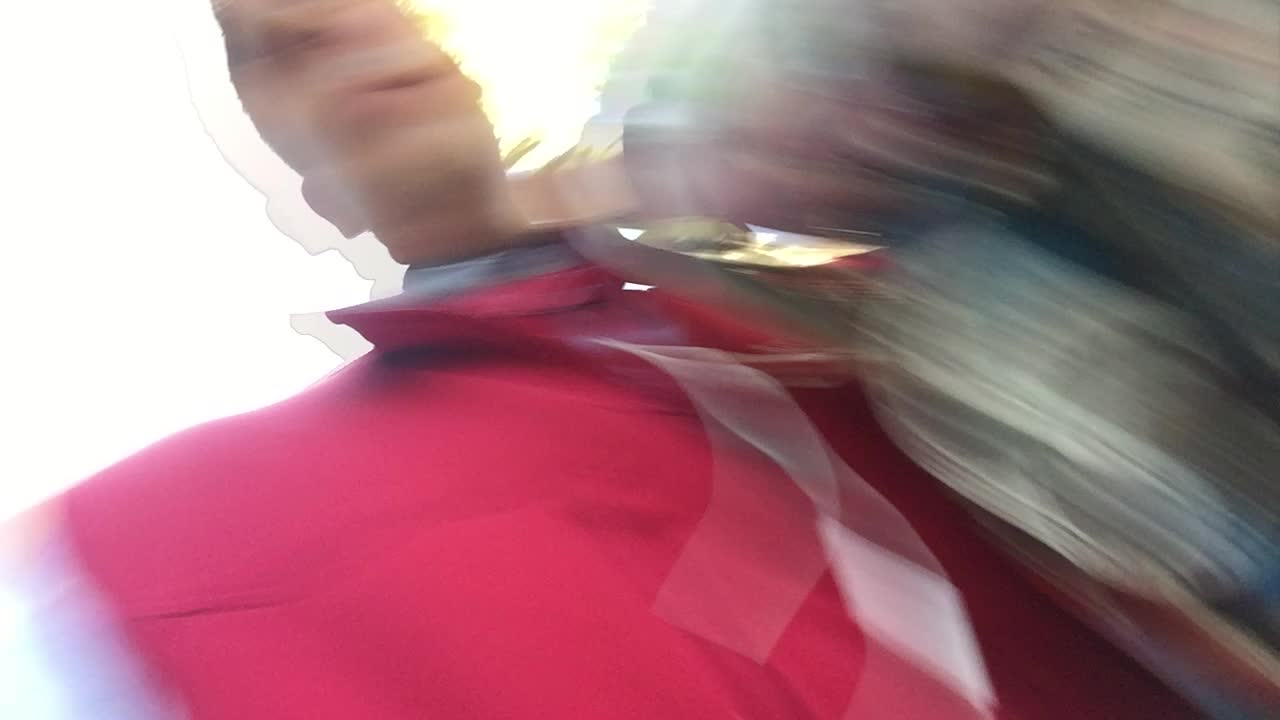In this blurry image, a person is captured in mid-motion, rendering their features indistinct. The individual appears to be wearing a button-up dress shirt, topped with a vibrant pink-magenta suit jacket, and a tie. Their hand is raised to their neck, seemingly attempting to loosen or remove the tie. The motion blur significantly obscures finer details, making it challenging to identify specific aspects of the scene or the person's identity.